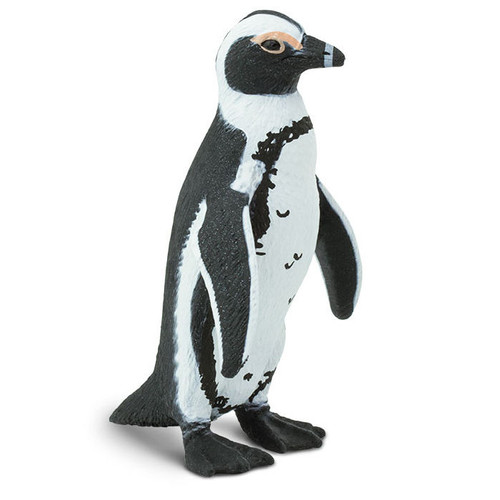The image features a penguin standing on a solid white background, devoid of any text or additional elements. Centered in the frame, the penguin is shown in a right side profile with its black beak pointing to the right from the viewer's perspective. The penguin’s head is predominantly black on the right side, but a distinctive white stripe runs along the right edge of the face. Notably, there's a pinkish hue outlining and just above the eye, which is black. The beak is primarily black with a subtle white circle around it.

The penguin’s body showcases a stark contrast between its white belly and black back, flippers, feet, and tail. The front flippers have a white outline, accentuating their black centers. Although the stomach is mostly white, it is dotted with small black specks. The penguin’s stance casts a subtle shadow, reinforcing the clean, minimalistic look of the composition, which emphasizes the penguin against the unadorned background.